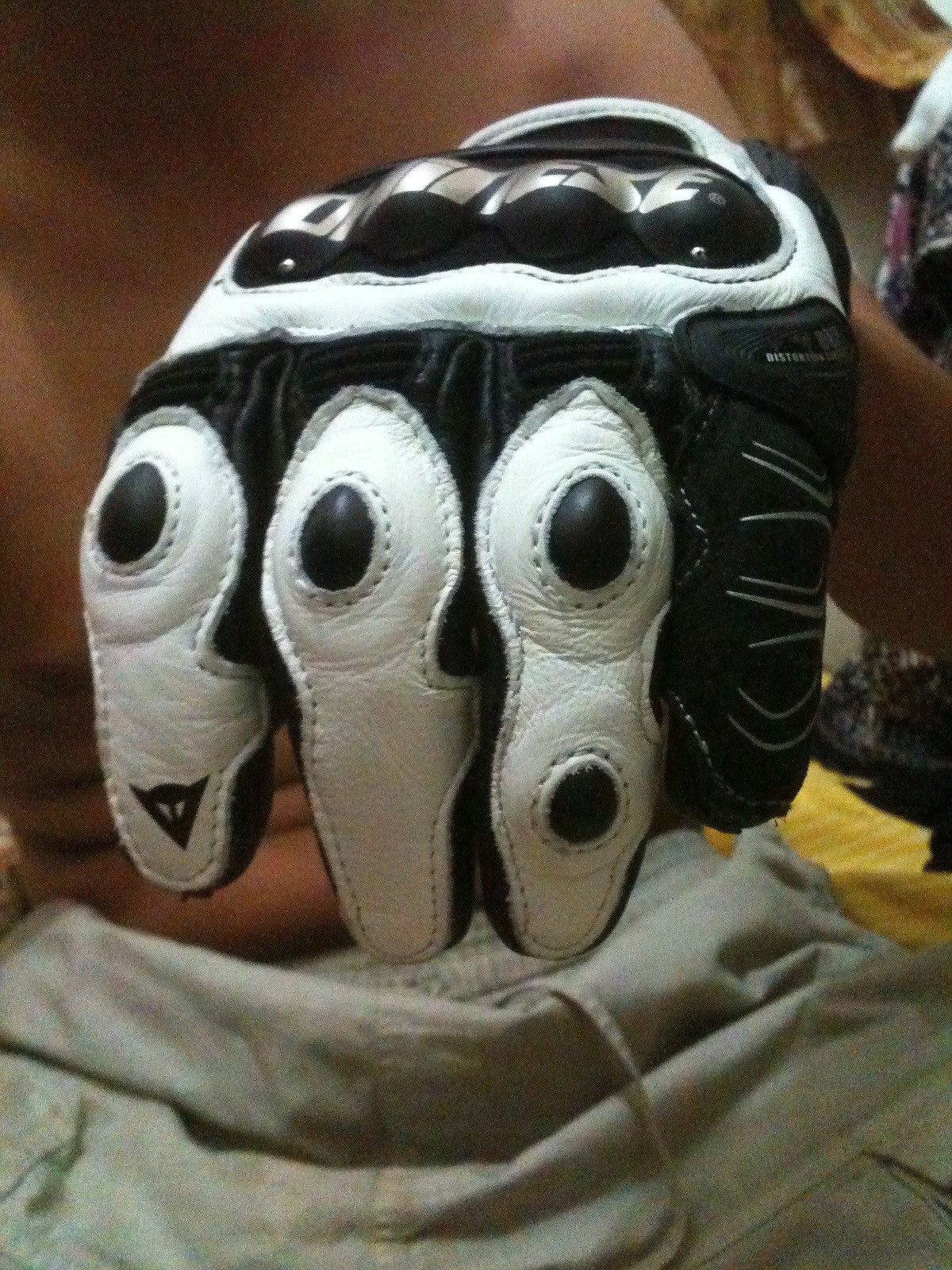The image features a close-up of a black and white hockey glove being held up by a shirtless man wearing gray sweatpants that are folded over. The glove showcases three white fingers and one black finger, with black tips towards the knuckles. It also has distinctive black circular areas towards the wrist, bordered in white. A prominent triangle icon is visible on the index finger. The glove's intricate details include pointed padding on the knuckles and finger bends, and silver tabs around the top. The man’s chest and a partial view of his arm are visible in the background, with a glimpse of a wood floor on the right side of the photo. The focus on the glove places it centrally in the image, measuring roughly about five inches tall and six inches wide.